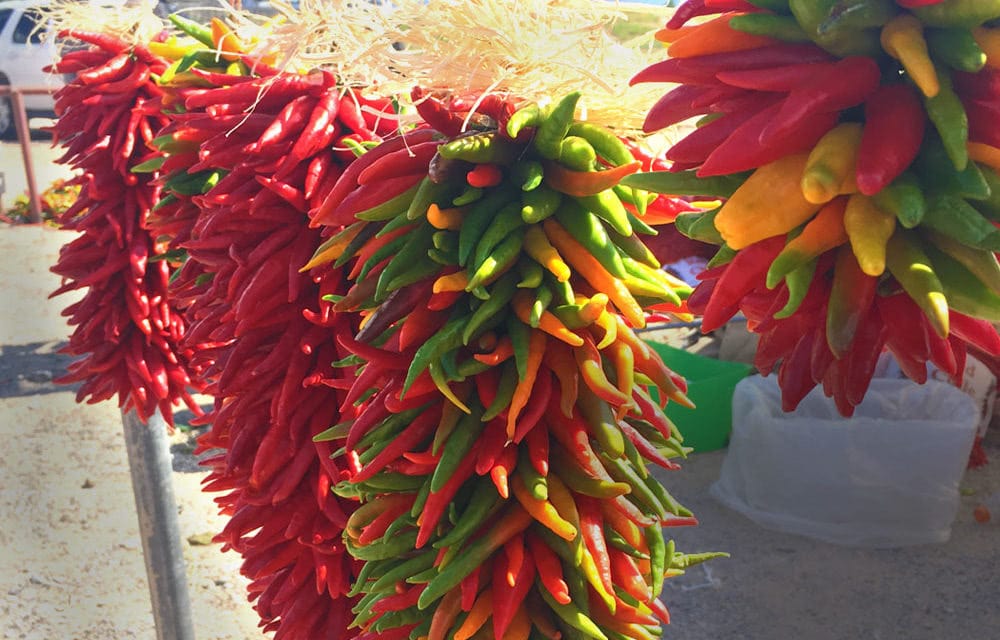This vibrant outdoor scene captures a display of long, pointy chili peppers at a market, intricately woven and stacked in vertical columns. The photo, taken on a sunny day, features several bunches of chilies hanging tightly together like bouquets. The foremost bunch at the center includes a vivid mix of red, green, yellow, and orange peppers, showcasing their varying stages of ripeness. Surrounding this central bunch are primarily red chili displays, with some featuring hints of green and yellow. A distinctive red chili, about a foot and a half long, hangs prominently in the background.

The background of the image reveals a sunny dirt ground with scattered metal fencing and posts. A white SUV is visible parked behind a concrete abutment, and a trash can with a white trash bag stands nearby. To the left of the peppers, a possible brick staircase or structure can be seen, along with a glimpse of yellowish greenery. The right side of the image shows a bucket with plastic in it, likely for collecting the chilies, placed on a cement walkway.